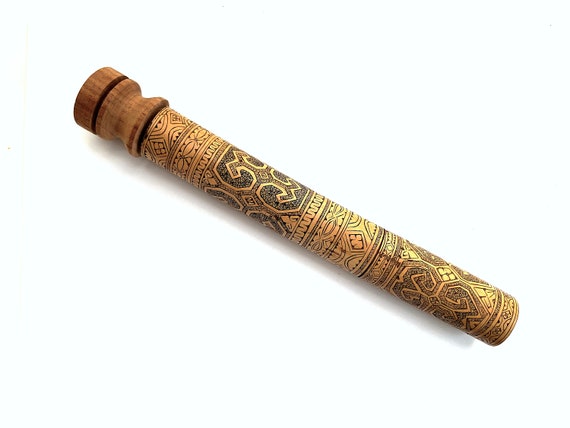The image features a long, thin, cylindrical wooden object that resembles a fancy pen casing or possibly an ancient scroll. The object is predominantly wood-colored with a darker wooden cap at the top, marked by a black ring around it. This cap includes a notch cut out underneath, likely for better grip. The main body of the cylinder showcases an intricate, ornate design characterized by delicate line art in black ink. The patterns vary along the length, with detailed sections including a light pink background near the top and a gray section with black dots and a yellow emblem in the center. As the intricate black patterns continue toward the bottom, the cylinder emits a yellowish tint. The entire object is set against a mostly white background, casting a distinct shadow to the left and beneath it, which is darker and emphasizes the object's three-dimensional form.